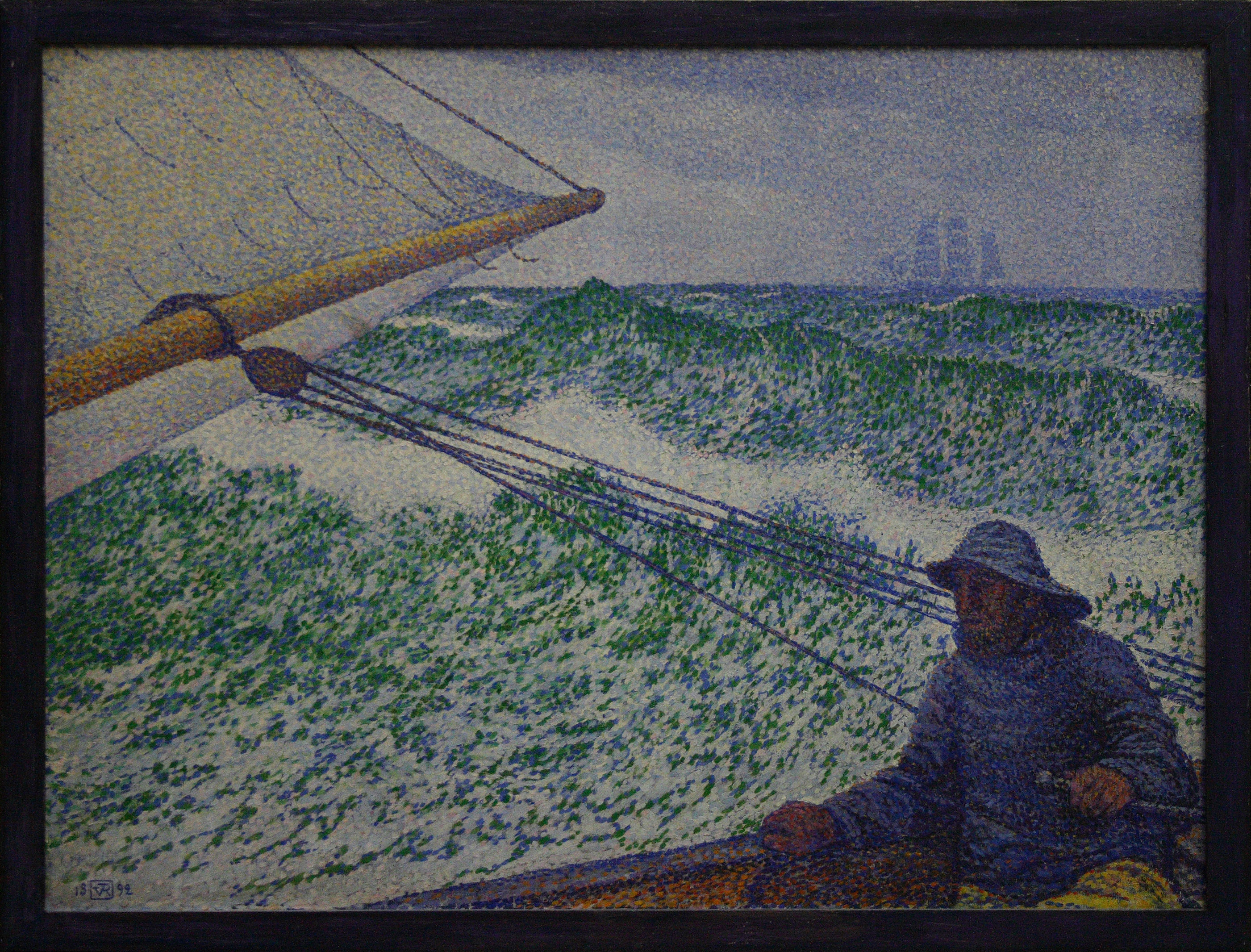This painting, created in a pointillism style using small dots to form the image, depicts a dramatic scene of a sailor navigating through a tumultuous sea during a violent storm. Positioned in the bottom right corner, the bearded sailor, a white man, is dressed in traditional rain gear—a blue hat, blue coat, and yellow pants—suggesting he's well-prepared for the wet conditions. With his left hand, he grasps a rudder, steering his smaller sailboat. The boat's sail, a prominent white canvas, is supported by numerous ropes leading to a mast, emphasized by the muted brown boom that holds it aloft. The setting is striking with towering, vibrant green waves that appear 50 to 60 feet high, casting the sea into an angry, formidable presence. In the distance, barely visible through the fog, lies the outline of a three-masted schooner, hinting at the broader maritime context. The sky above is a deep blue, accented with soft white lines, adding to the overall impressionistic and muted color palette dominated by grays and blues. The scene captures the essence of struggle and perseverance against nature's fury, evoking the 1800s era of seafaring and fishing.